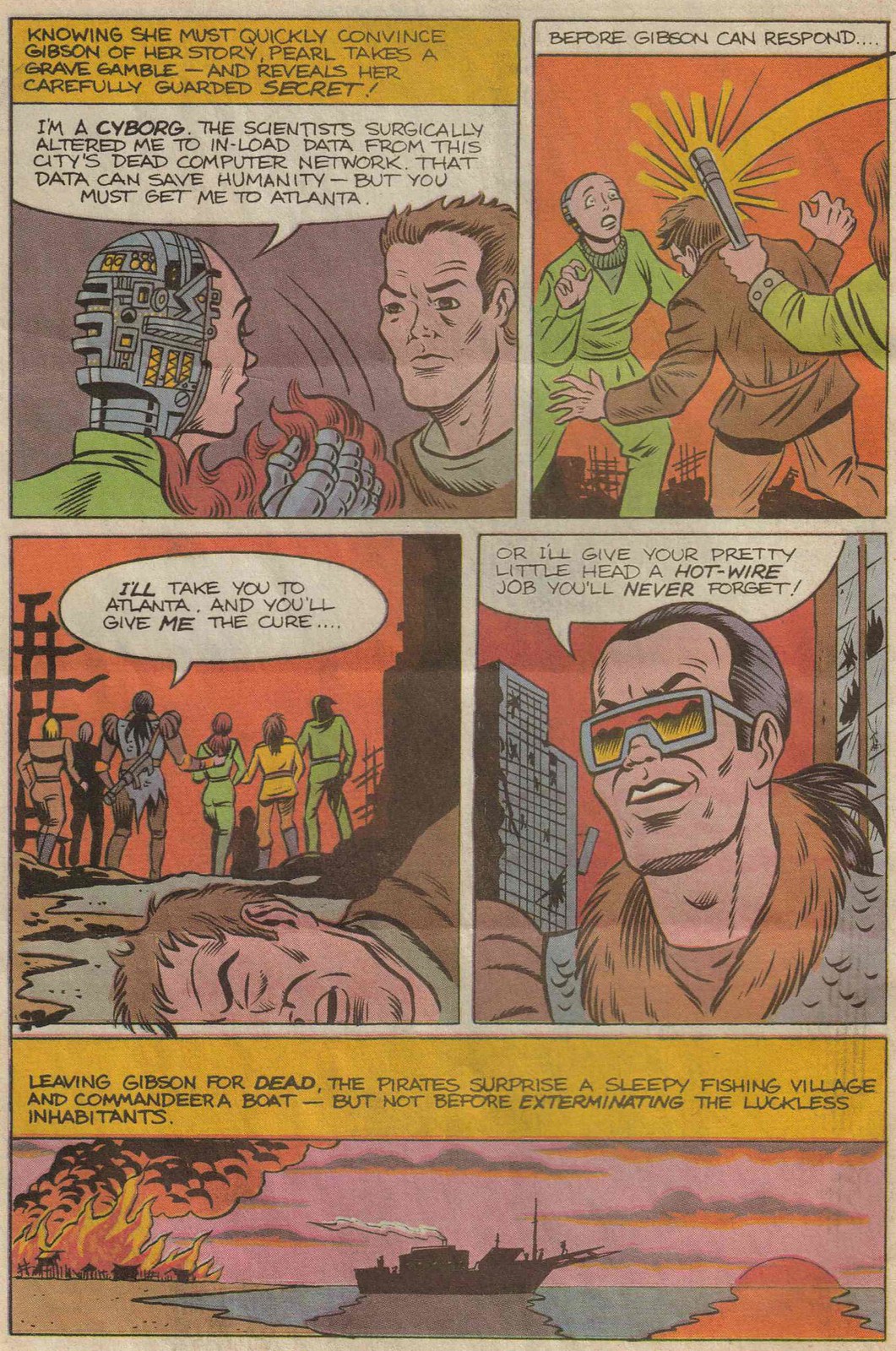This comic page is divided into five panels, with two on the top third, two in the center, and one spanning the bottom. In the top left panel, a gold box narrates: "Knowing she must quickly convince Gibson of her story, Pearl takes a grave gamble and reveals her carefully guarded secret." Pearl, a cyborg with the back of her head exposing circuitry, metal plating, and yellow lights, tells a short brown-haired man, "I'm a cyborg. The scientists surgically altered me to inload data from this city's dead computer network. That data can save humanity, but you must get me to Atlanta." Before Gibson can respond, the adjacent top right panel shows a villain striking him on the back of the head as Pearl looks on with concern. The central left panel has the villain saying, "I'll take you to Atlanta, and you'll give me the cure," while Gibson lies unconscious on the ground, and Pearl is forcibly escorted by a group of people. In the central right panel, the villain, now wearing sunglasses, threatens, "or I'll give your pretty little head a hot wire job you'll never forget." The bottom panel, covering the entire width of the page, depicts a battleship in the ocean at sunset. On the right side of the scene, flames and smoke rise ominously from a raid, narrated by another gold box: "Leaving Gibson for dead, the pirates surprise a sleepy fishing village and commandeer a boat, but not before exterminating the luckless inhabitants."